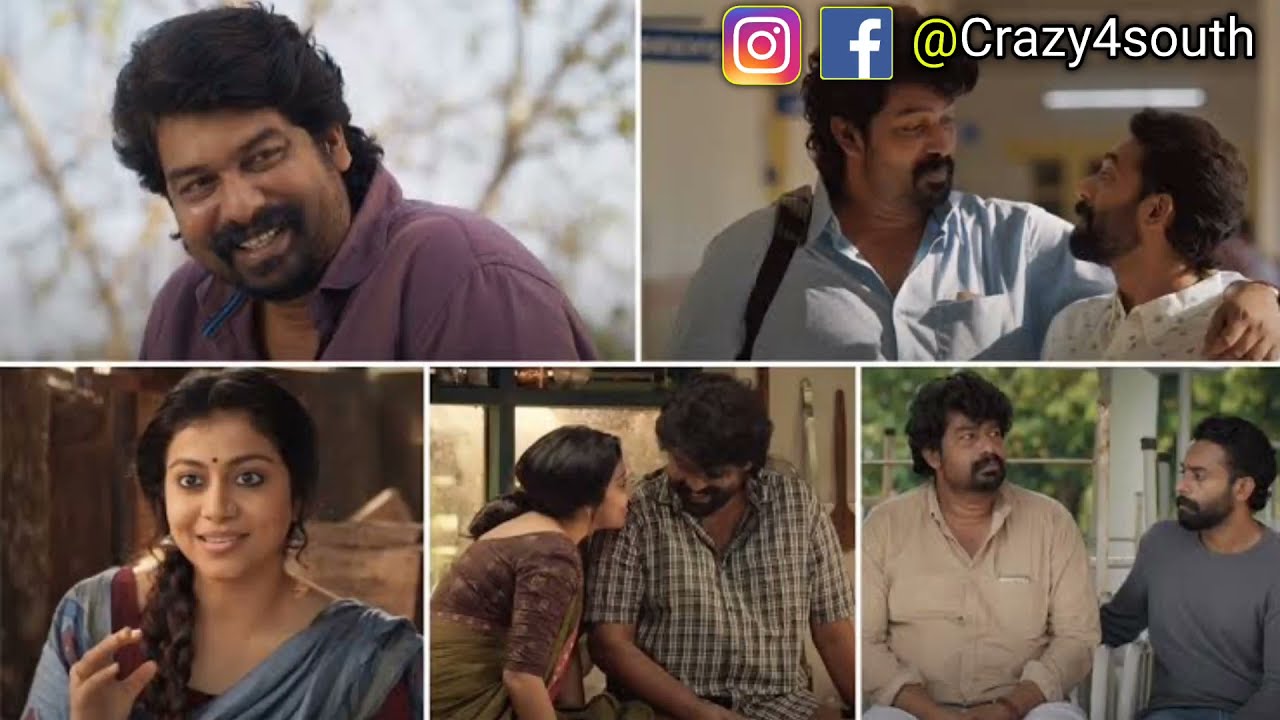The image is a collage of five photographs featuring an Indian man and various characters from what looks like either a Bollywood show or a social media series. 

In the top row, the left picture depicts a middle-aged, chubby Indian man with thick medium-length black hair and a black goatee, wearing a purplish eggplant-colored collared shirt. He is smiling with an outdoor backdrop of trees. Next to this, on the top right, is the same man in a blue button-down shirt standing with his arm around another man. This second man has black hair, a beard, and is wearing a white shirt with subtle patterns. Above them are Instagram and Facebook icons, alongside the handle "@crazy4south."

The bottom row includes three images. The first on the left shows an Indian woman with long braided dark hair, wearing a blue shawl and a burgundy shirt underneath, against a darker background. The center picture again features the man from above, but now in a green and white checkered shirt, sitting next to the same woman, both of them laughing. The final picture on the right shows the main man in a tan shirt standing beside a younger Indian man in a gray shirt, with a backdrop of green trees.

This detailed collection of images seems to capture moments from a social media series or a television show, emphasizing the main man's life and interactions with others.